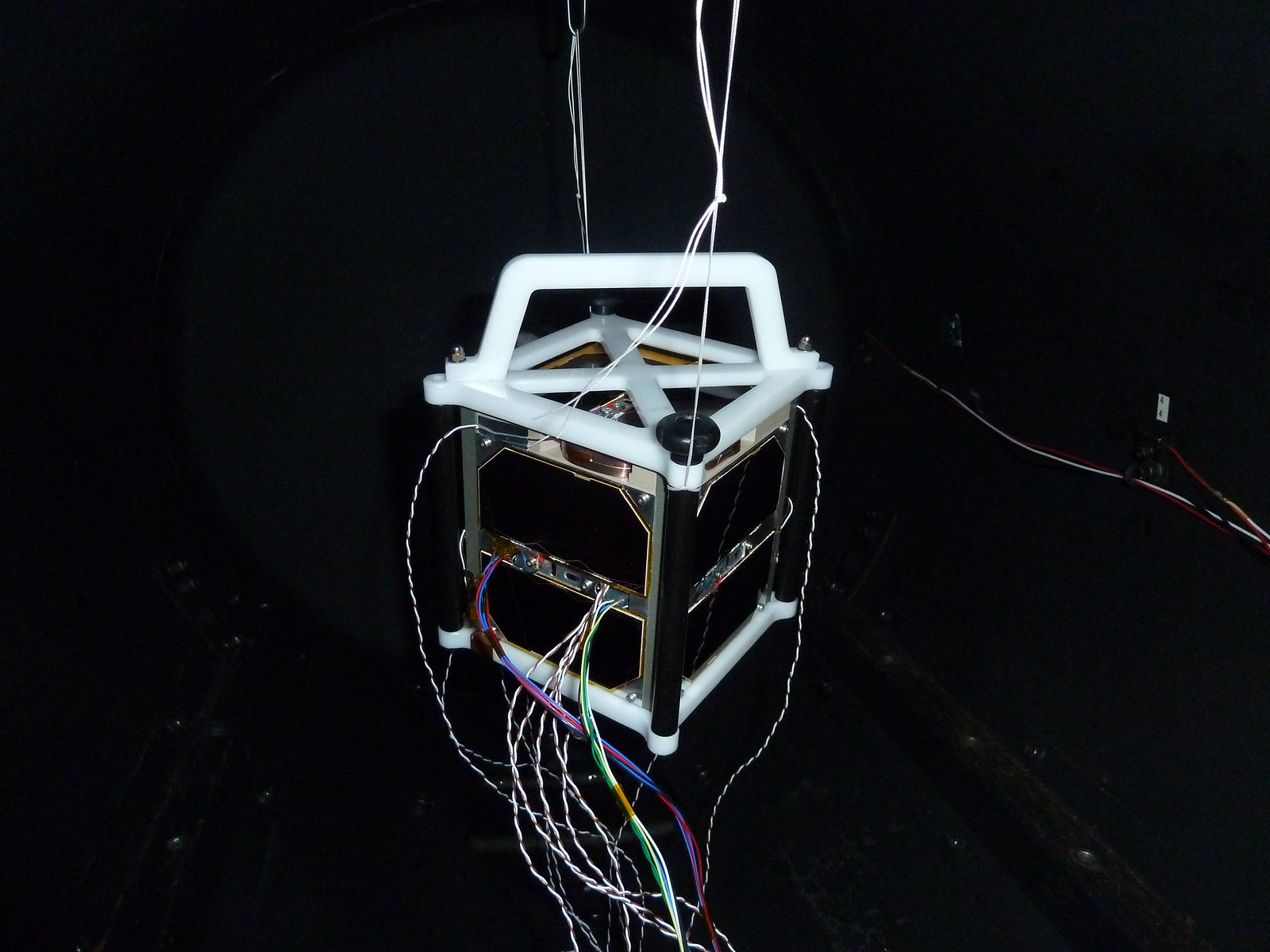In this darkened image, an electrical device is prominently featured, either hanging in the air or resting on a black surface. The device is framed within a dark box made from square piping, with a white plastic top and bottom that each contain a diagonal white handle forming an X-shaped support. The device's edges, constructed from silver metal, are fastened with long black bolts at each of the four corners. An array of colorful wires—green, pink, blue, white with black or brown-gray stripes, purple, red, and yellow—are connected to various parts of the device, including the top, middle, and bottom. Additional white strings and wires also secure it, suggesting the apparatus is being suspended. The main colors present in this detailed setup are black, white, and dark green, creating a striking contrast against the black background.